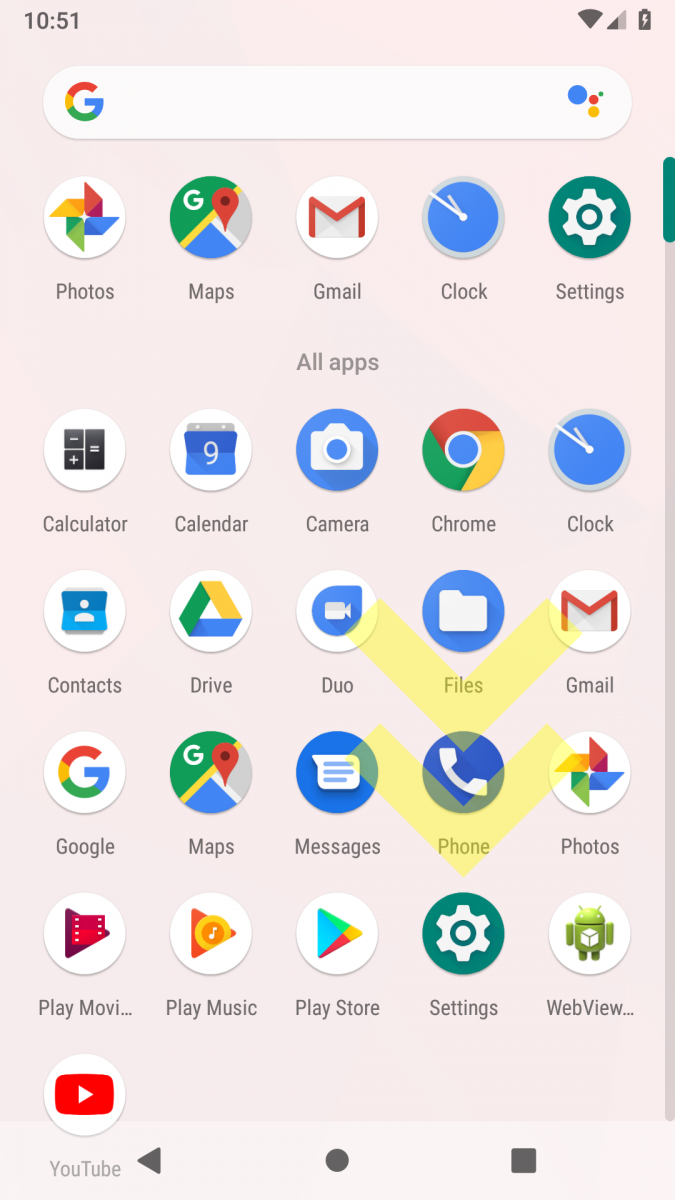A detailed and organized image description:



The image displays a phone screen captured at 10:51 PM, showcasing a fully charged battery. The primary interface is Google-centric, emphasizing various Google services and apps. Here’s a detailed breakdown of the apps visible on the screen:

1. **First Row (left to right)**:
   - **Google Search**: An all-purpose search bar for browsing the web.
   - **Google Photos**: An app dedicated to storing and organizing photos.
   - **Google Maps**: Navigation and mapping service.
   - **Gmail**: Email service by Google.
   - **Clock**: Standard clock app.
   - **Settings**: The device settings icon.

2. **Second Row (left to right)**:
   - **Calculator**: Basic calculator app.
   - **Calendar**: Scheduling and event management.
   - **Camera**: The phone’s camera application.
   - **Google Chrome**: Google’s web browser.
   - **Clock**: Another clock icon, suggesting a potential shortcut or additional clock-related functionality.

3. **Third Row (left to right)**:
   - **Contacts**: Phone book for storing contact information.
   - **Google Drive**: Cloud storage service.
   - **Duo**: Video calling app by Google.
   - **Files**: File management app.
   - **Gmail**: An additional shortcut to the Gmail app.

4. **Fourth Row (left to right)**:
   - **Google**: Another shortcut to the Google search app.
   - **Google Maps**: Another shortcut to Google Maps.
   - **Messages**: Text messaging app.
   - **Phone**: Dialer for making calls.
   - **Google Photos**: Another Google Photos icon.

5. **Fifth Row (left to right)**:
   - **Play Movies**: Google’s app for purchasing and streaming movies.
   - **Play Music**: Google’s music app.
   - **Play Store**: Google’s app marketplace.
   - **Settings**: Another settings icon, highlighting the repetition.
   - **Web View**: Likely a shortcut for web browsing or development purposes.
   - **YouTube**: Video streaming service.

Additionally, a noticeable yellow arrow is pointing downwards, connecting Duo and Gmail, and extending to the Phone icon in the fourth row. This visual element suggests some guidance or emphasis on these apps.

The screen features numerous repetitive icons, including multiple instances of Gmail, Google Maps, Clock, Google Photos, and Settings, which stands out as particularly unusual for a regular phone setup.